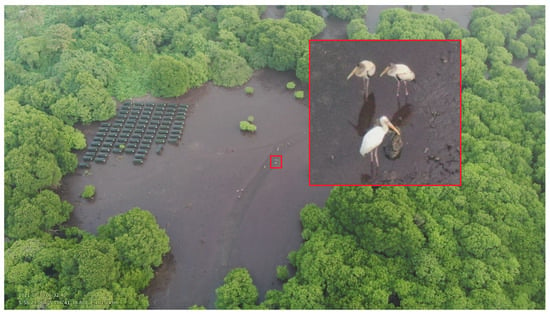This is an aerial view of a lush, green forested area centered around a wetland pond, rich in biodiversity. In the pond, numerous small tree islands and white specks are visible, with one speck highlighted by a red square. Within this red square, an enlarged close-up reveals three shorebirds with long legs and distinctive long bills, likely spoonbill herons, wading in the water, foraging for food. Surrounding the pond are rows of peculiar small structures, possibly steel tanks or ecological installations, arranged neatly in lines about ten deep and ten wide, occupying a small fraction of the water area. The area overall resembles an estuary bordered by mangroves, suggesting a saltwater ecosystem, typically found along coastal regions such as the Atlantic or the Gulf Coast.